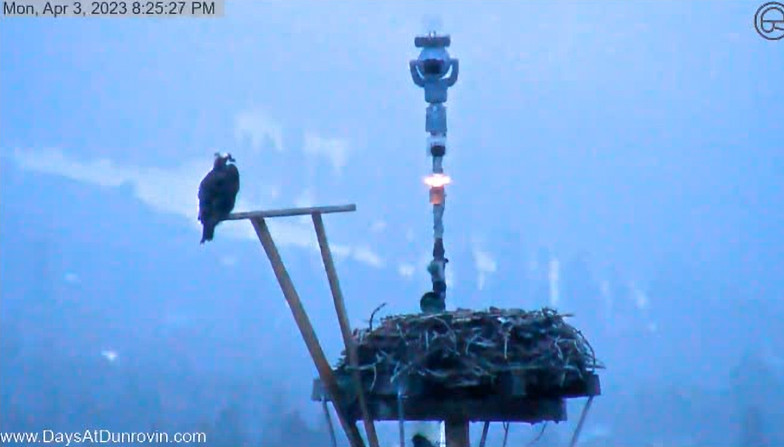This rectangular photograph, taken outdoors on Monday, April 3, 2023, at 8:25:27 PM, features a slightly foggy and out-of-focus scene with a light blue hazy background. In the upper left-hand corner, a gray bar displays the date and time stamp, while the lower left-hand corner has the website www.daysatdunroven.com in white letters. Dominating the image is a man-made platform, likely part of a tall tower, with hay or grass resembling a large bird's nest. Extending from the platform are several lines, possibly wires, which travel out of the frame. Beneath the platform, a portion of a pole is visible, continuing downward beyond the scope of the photograph.

To the left of the nest, two vertical rods rise about two feet above the platform, connected by a horizontal piece that serves as a perch. A large bird, possibly an eagle or an osprey, is perched on this horizontal piece. The bird is primarily black with distinctive white markings on its head and cheeks. In the background, beyond the platform, stands another pole topped with a rounded object that appears to be a CCTV camera. This pole features a light emitting from a section beneath the camera, contributing to the slightly foggy ambiance of the scene.